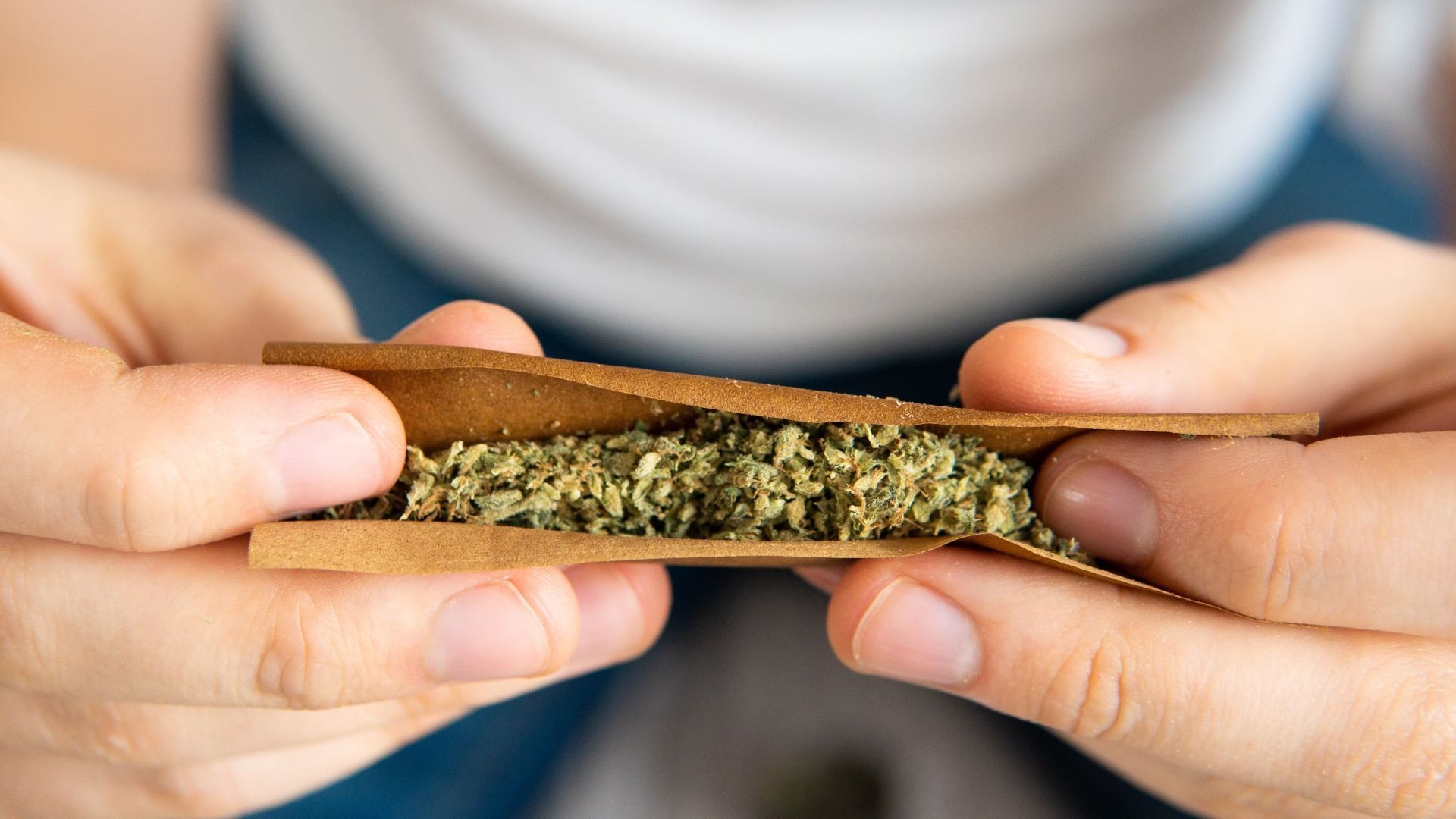The photograph captures a detailed close-up of a person in the midst of rolling a marijuana joint. The individual, who appears to be male and is wearing a white shirt and blue jeans, holds a thin, brown rolling paper filled with finely chopped, light yellow and green marijuana leaves. The paper, not yet fully wrapped, is being skillfully manipulated into a cylindrical shape. Both hands are engaged in the process: the left hand with three fingers visible, one of which is inside the paper, and the right hand with all four fingers and the thumb clearly holding the other end of the paper. The person's fingers are positioned meticulously to curl the paper into the familiar joint shape, demonstrating a moment just before the joint is completely rolled.